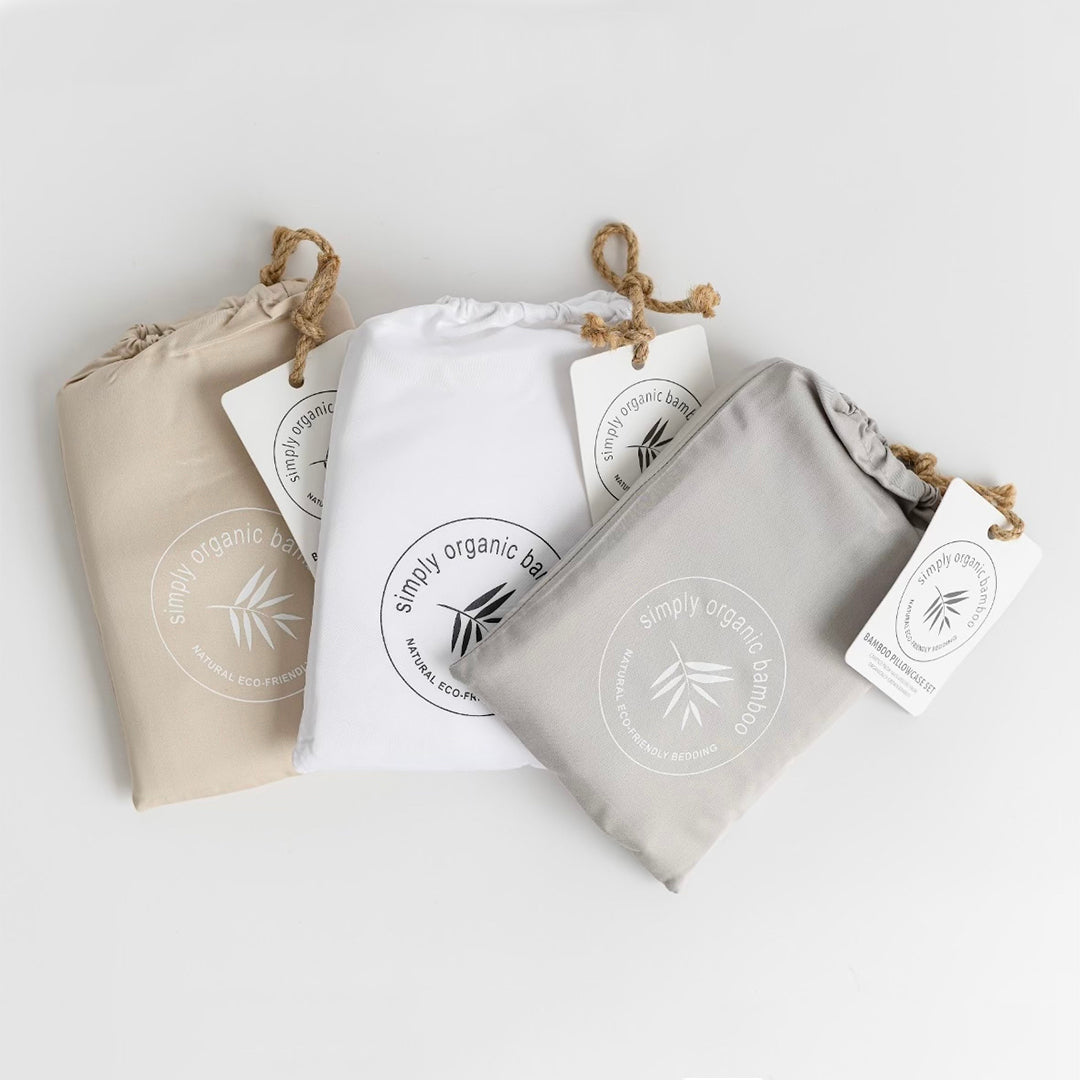This bird's-eye view photograph captures a neatly arranged trio of drawstring pouches on a solid white tabletop. Each pouch is a different color—tan, white, and gray—and they partially overlap each other in a fan-like arrangement. The drawstring of each bag, made from rustic twine, secures a white tag branded with the same logo found on the bags themselves. This logo features a circular design with a stylized bamboo leaf, and the text "Simply Organic Bamboo." The logo also includes a smaller tagline that reads "Natural, Eco-Friendly Bedding." The tags indicate that these bags are part of a “Bamboo Pillowcase Set," reinforcing the brand's commitment to eco-friendly, sustainable products. The consistent design and branding underscore the cohesive visual identity of Simply Organic Bamboo.